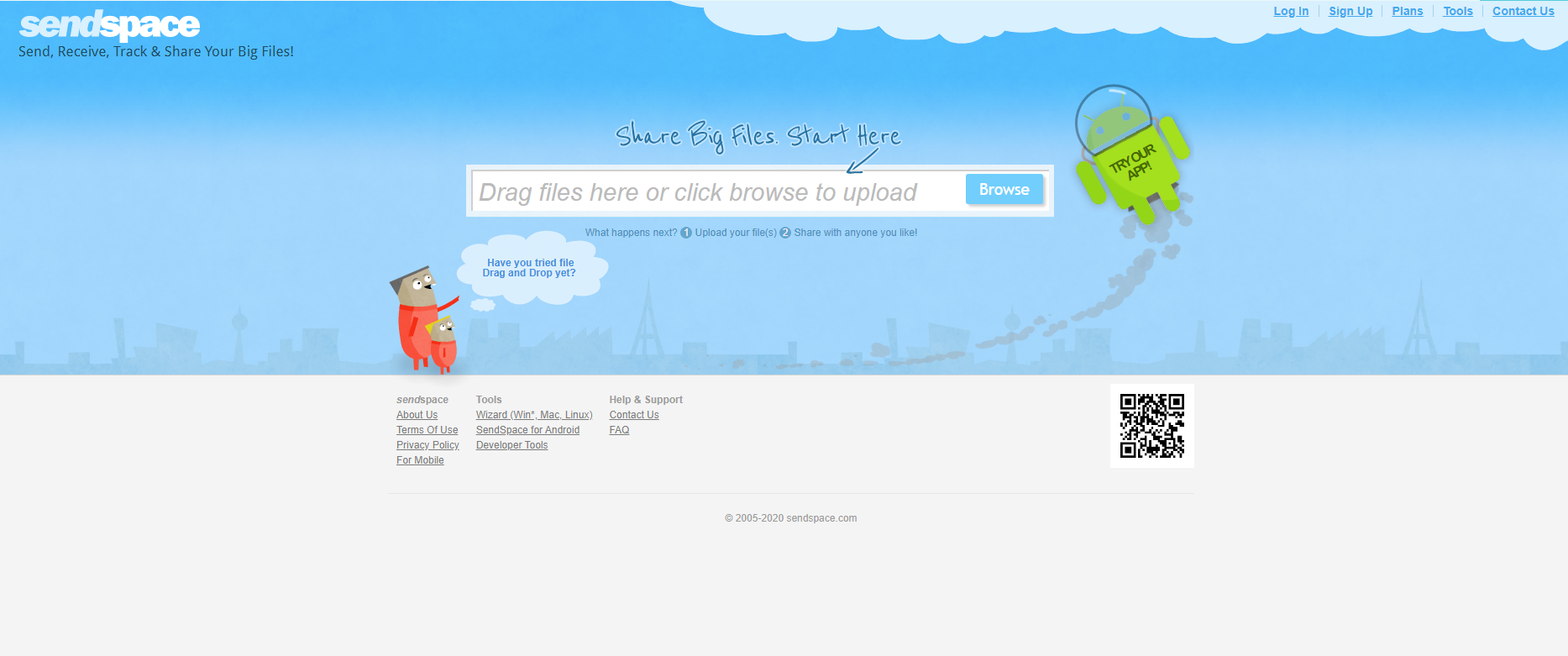Description: A website start page, visually divided horizontally into two color sections. The upper half features a blue sky background with a cityscape silhouette along the horizon. In the top left corner, the Send Space logo is displayed above the tagline "Send, Receive, Track, and Share Your Big Files" in black type. Moving right from the center to the top-right corner, fluffy clouds adorn the background, while navigation links such as Login, Sign Up, Plans, Tools, and Contact Us are neatly aligned.

In the center of the blue section is a prominent white rectangular box inviting users to "Drag Files Here or Click Browse to Upload," with a blue Browse button on its right side. Above this box, in a playful, handwritten font, the text "Share Big Files Start Here" is accompanied by an arrow pointing toward the box. Two cartoon characters, resembling a man and a child in orange suits, are positioned to the bottom left of the box, with the child asking, "Have You Tried the Drag and Drop Yet?" The man points towards the box, guiding user interaction.

To the right of the white box, an Android icon, donned in a space helmet, promotes the mobile app with the text "Try Our App."

The bottom half of the page features a light gray background. On the mid-left side are essential links for About Us, Terms of Use, and other detailed options. To the mid-right side of this section lies a QR code, providing an additional way for users to access site features.